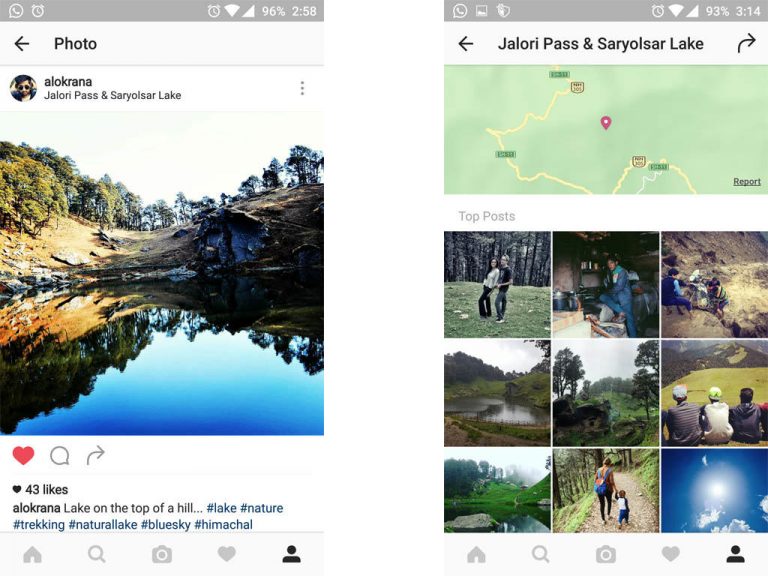In this image, we see two separate cell phone screens side by side. The screen on the left resembles an Instagram post. At the top left, there are icons for WhatsApp, a clock, and an alarm, followed by a Wi-Fi connection icon, a 96% battery life indicator, and the time displayed as 2:58 PM against a gray background. Below this is a photo post that includes an arrow pointing left. The post is from a user named L.O.Crana and is captioned "Jalori Pass and Sari Losar Lake." The image within the post features a picturesque lake set against a backdrop of land. Underneath the image, there are interactive icons: a red heart, a comment bubble, and a share arrow. Below these icons, it's noted that the post has 43 likes with the caption "lake on top of the hill" followed by blue hashtags. At the very bottom, the screen has five app navigation icons: a home screen, a search magnifying glass, a camera, a heart, and a user profile symbol.

The screen on the right shares the same five navigation icons at its bottom. The top of this screen includes the same basic status icons as the left screen, but the time now reads 3:14 PM, and the battery life is at 93%. Directly beneath these icons, the screen displays the location "Jalori Pass and Sari Losar Lake" again. The main part of the screen features a map showing the location. Below the map is a section labeled "Top Post," which displays a grid of nine square images, each highlighting various nature scenes from the same location.